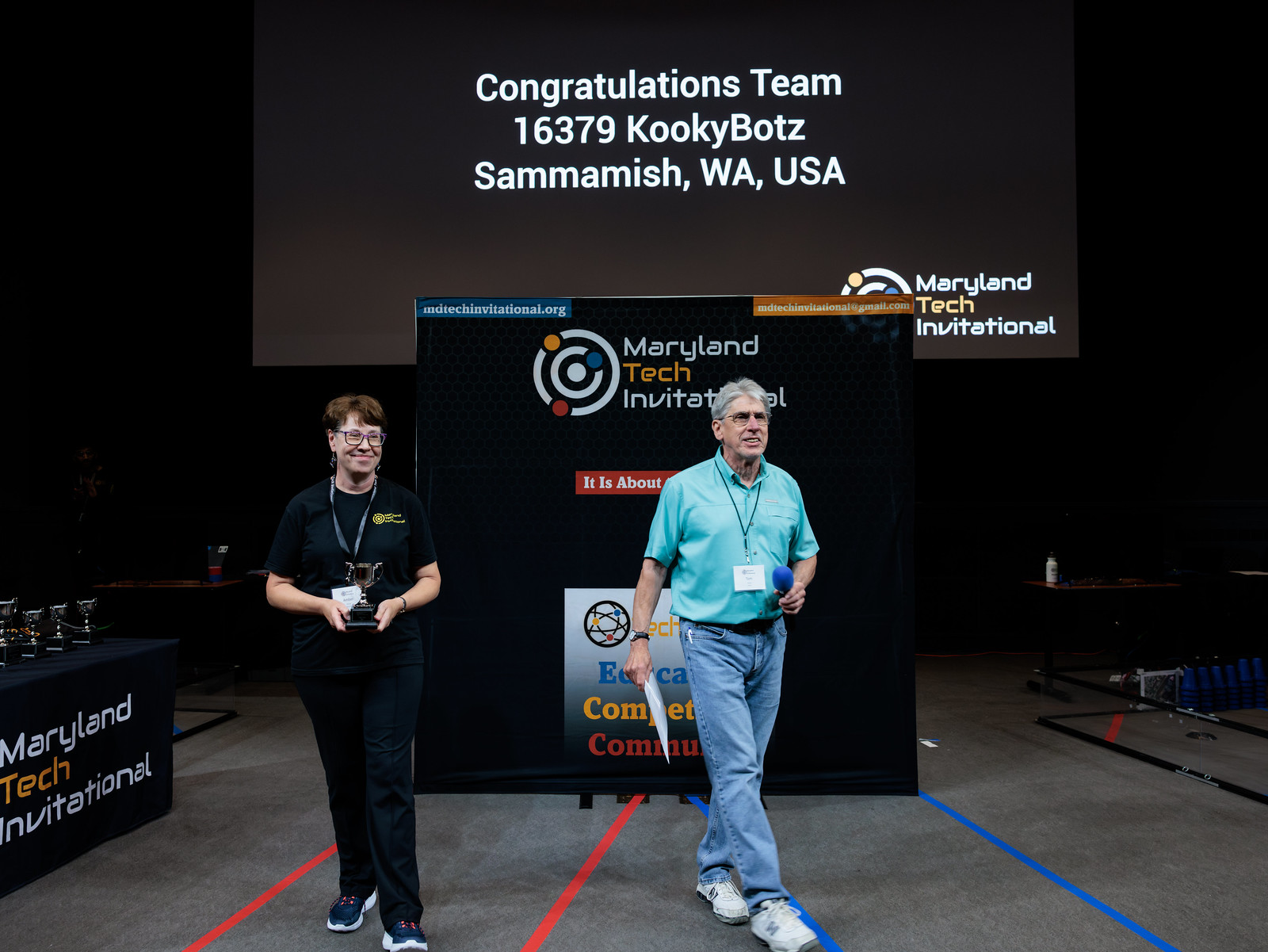The photograph captures a moment at the Maryland Tech Invitational, taking place within an indoor convention center. In the background, a large screen displays the message: "Congratulations Team 16379 Cookie Bots, Sammamish, Washington, USA." To the right of the text, it reads "Maryland Tech Invitational," indicating the event's competitive nature. 

In the foreground, two individuals are prominently featured. On the right stands an older man with gray hair wearing a green (or turquoise) shirt, blue jeans, and white tennis shoes. He carries a microphone with a blue top in his left hand and a piece of paper in his right, where he also sports a watch. A black lanyard with a white tag hangs around his neck. Standing to his left is a woman with red hair and black glasses, dressed in black attire and black tennis shoes with distinctive red shoelaces. She is holding a trophy and smiling, suggesting she’s possibly announcing the winner or presenting the award.

The setting features gray carpeted flooring with visible blue and red lines marking different sections. A table on the left holds additional trophies, underscoring the achievement-oriented atmosphere of the event. Both individuals appear to be moving towards the camera, beaming with pride and joy, encapsulating the celebratory mood of the occasion.